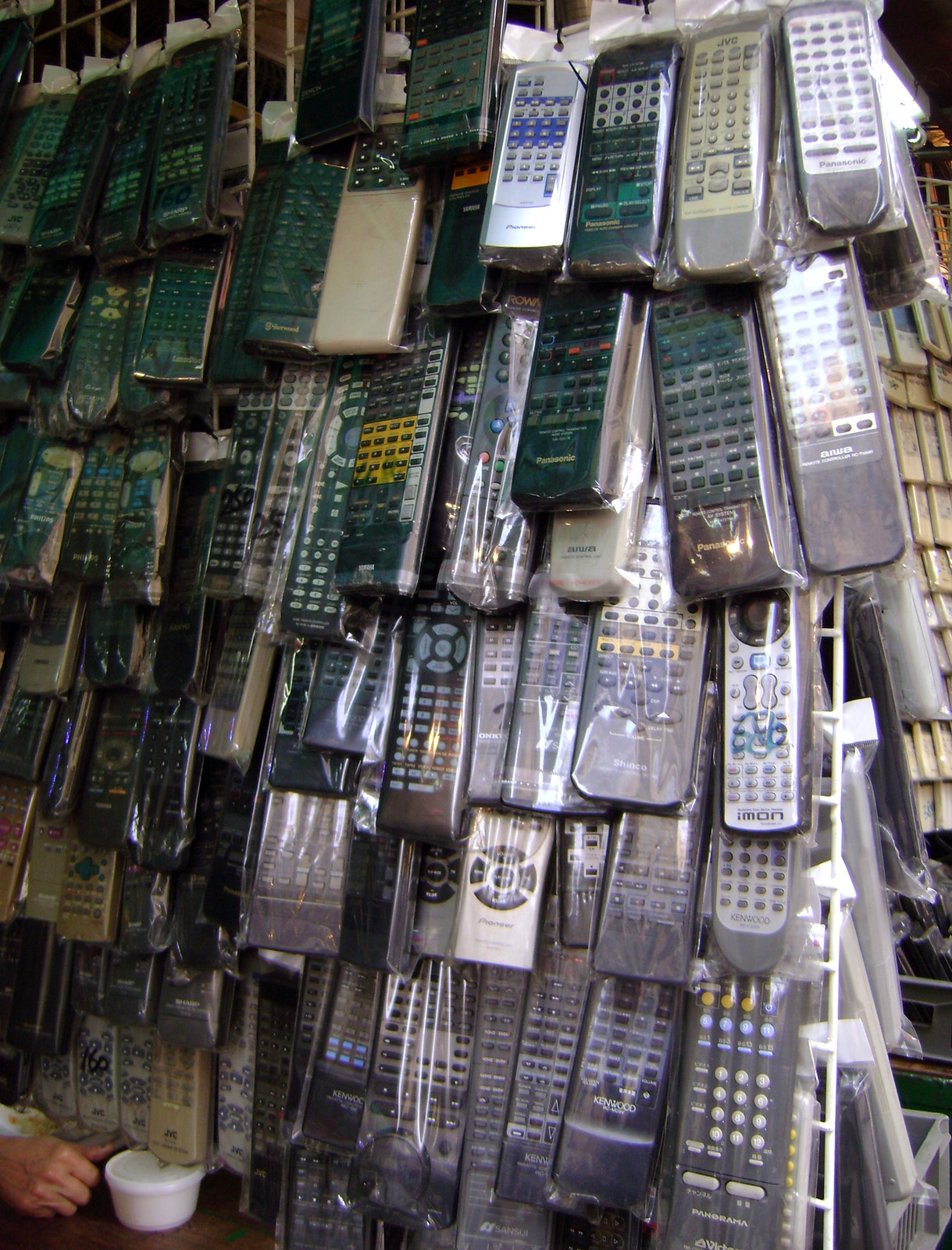The image depicts a store display consisting of a white wire rack covered with numerous TV remote controls, all individually wrapped in plastic bags. The remotes, varying in size, shape, and color, hang neatly in multiple rows, with many featuring buttons in an array of colors such as black, blue, green, and white. Positioned in the bottom left corner is a person's Caucasian right hand extending towards a round white container, possibly reaching for a coffee cup. The remotes include different models and brands, although most are either black, silver, or gray. This detailed assortment of remotes showcases everything from those with numerous buttons to simpler designs, all organized without any store name visible. The intriguing variety and meticulous arrangement suggest that this shop specializes in selling TV remotes, some dating back several years.